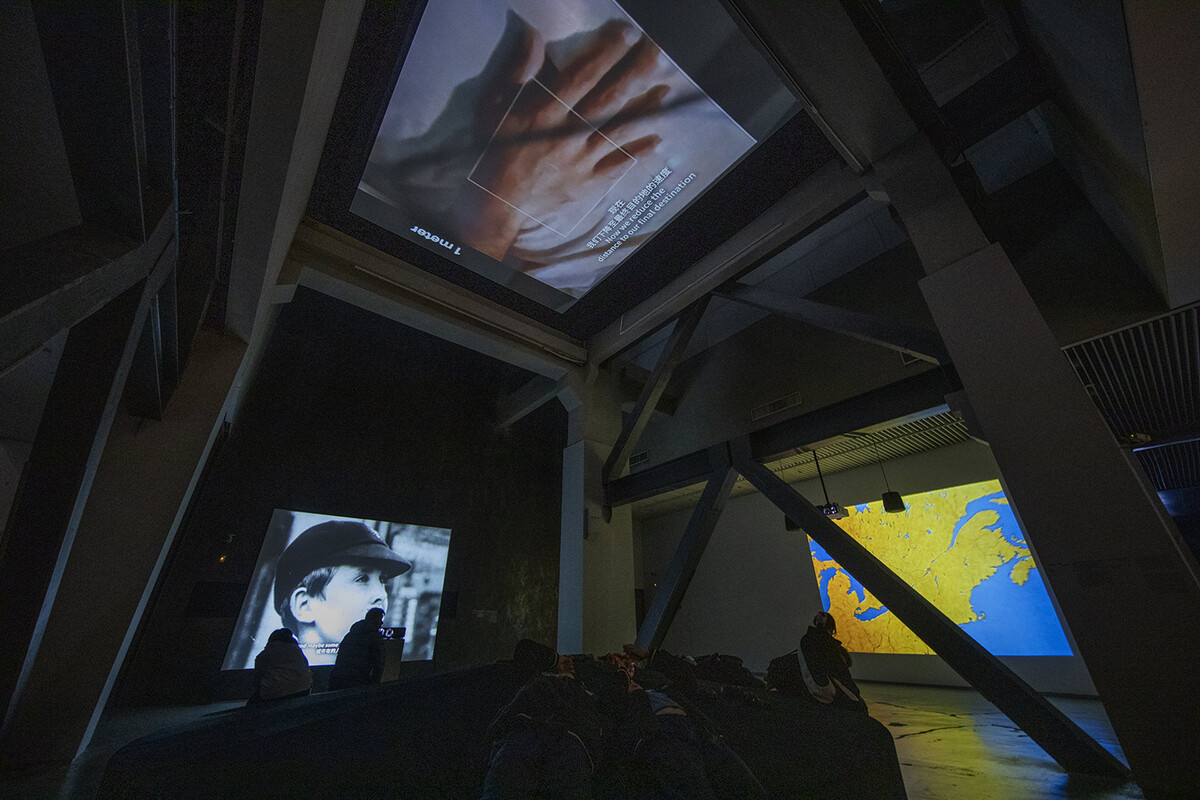In this dimly lit and enigmatic scene, we find ourselves inside a structure characterized by earthy brown walls and wooden support beams, lending the atmosphere an aged, almost rustic quality. The interior space is sparsely illuminated, making it challenging to discern finer details. Scattered throughout the room, there are several people; their indistinct figures suggest a variety of postures, with a few individuals lying on their backs atop bed-like structures draped in black covers, while others are seated upright.

Suspended overhead, a TV screen occupies part of the ceiling, contributing to the surreal ambiance. On one wall, there hangs a striking black-and-white image of a young boy donning a black hat, evoking a nostalgic, almost haunting presence. Another intriguing visual element is a hand with a white square outlined in its center, displayed prominently in the frame. Accompanying text, some of which appears to be in an Asian script, possibly Chinese, adds an element of international mystery.

On a different wall, a map delineates the outlines of the Northeast United States and Southeast Canada including the Maritimes, though it remains unlabeled and starkly blank, offering a stark contrast to the otherwise cluttered scene. This densely packed room, with its overlapping visuals and dark shadows, invites curiosity, leaving much to the imagination.